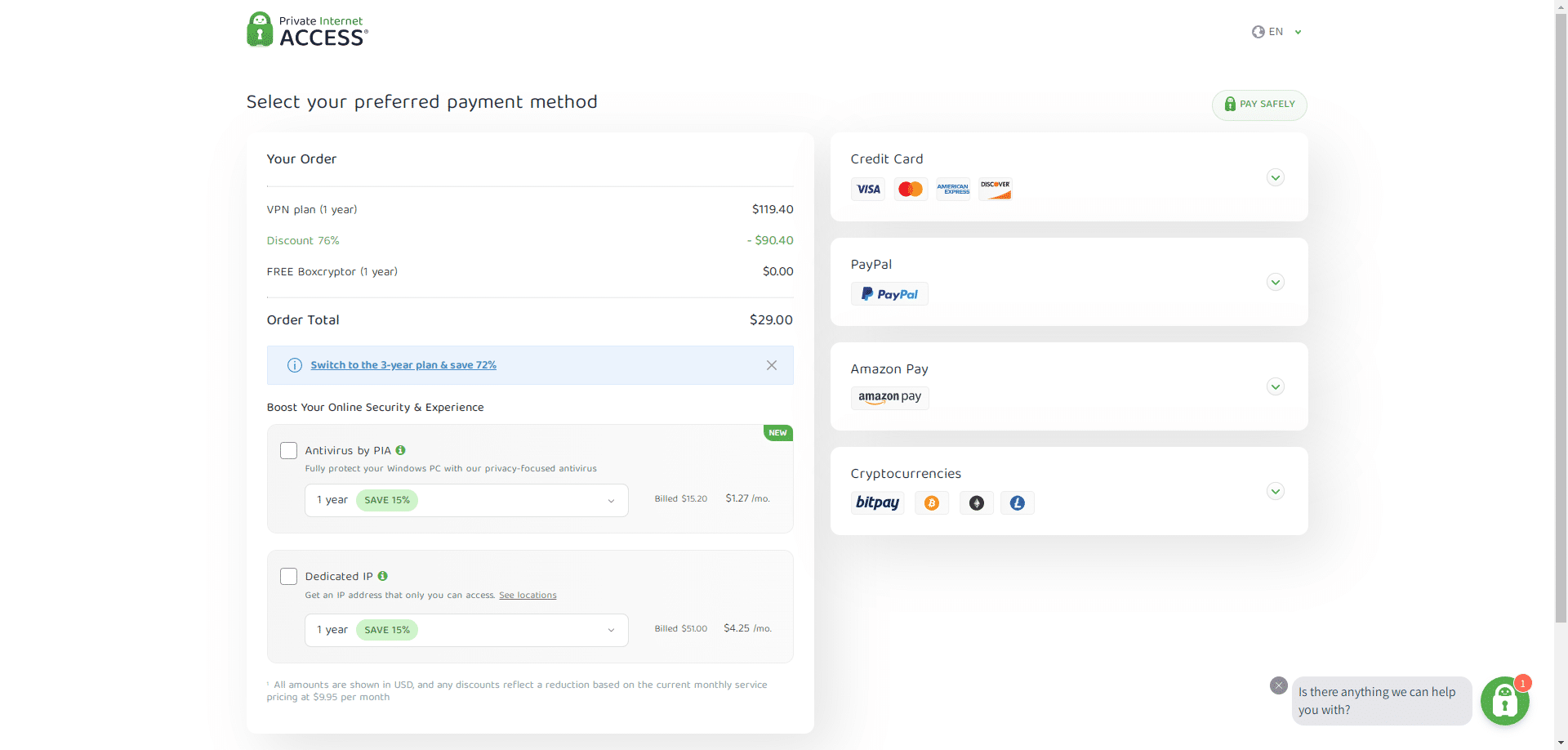A screenshot of a website's checkout page is displayed. At the top left section, the most prominent word "Access" is visible, followed by the instruction "Select your preferred payment method." Below this, a section titled "Your Order" is listed, mentioning "**VPN - One Year**" priced at **$119.40**. A discount is applied, stated as a reduction of **$90 or $60.40** (the exact amount is unclear), resulting in an order total of **$29.00**. Two add-on options are also available.

To the right, various payment options are arranged in boxes. The first box is labeled "**Credit Card**" and shows the logos for Visa, MasterCard, Discover, and American Express. The next section is labeled "**PayPal**," followed by "**Amazon Pay**," and the final section is titled "**Cryptocurrencies**," offering an array of payment methods for the purchase.